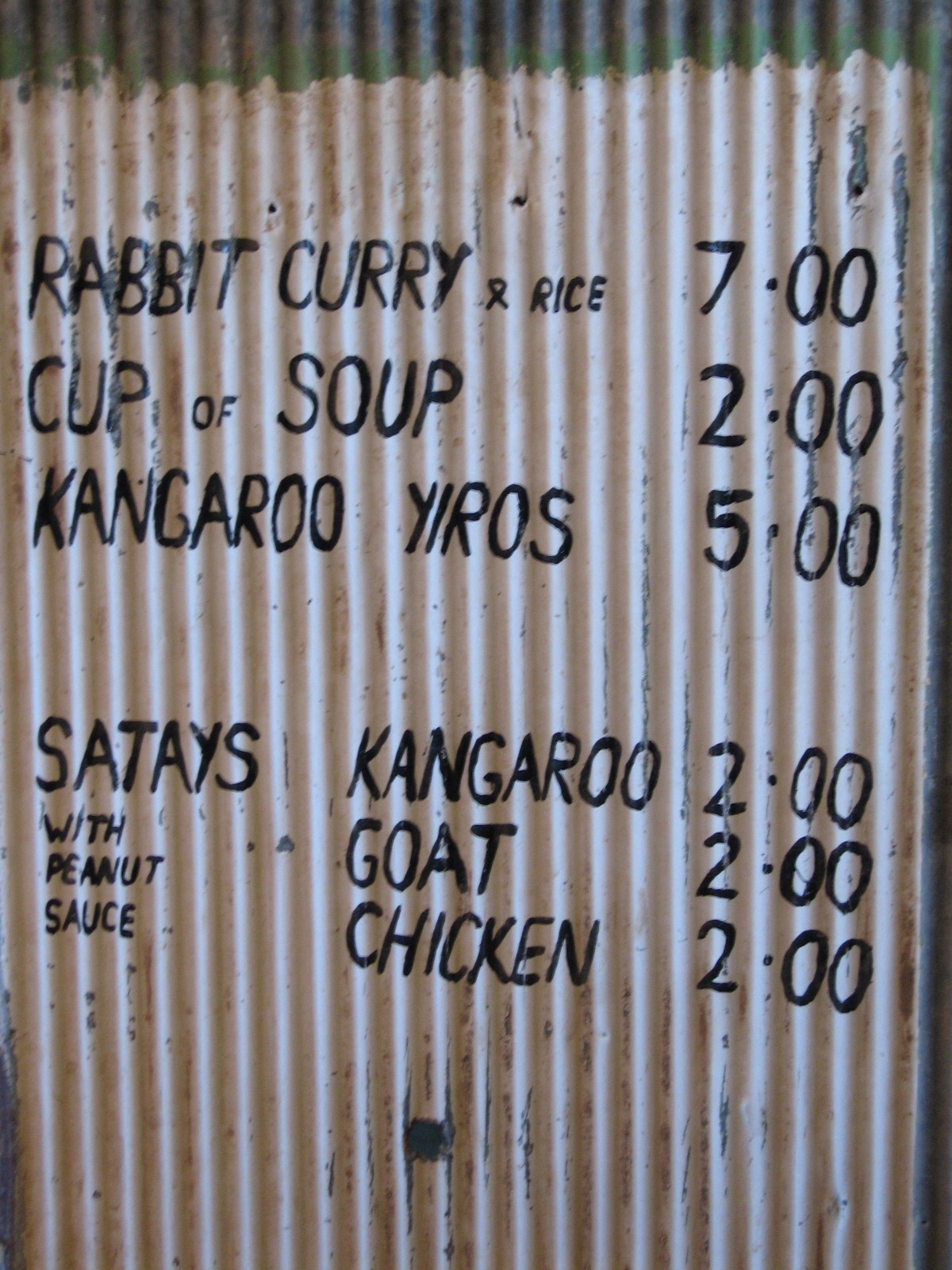The image depicts a rustic and simplistic menu that appears to be hand-painted on a piece of ribbed sheet metal. The menu lists the following options: "Rabbit Curry and Rice" priced at $7.00, "Cup of Soup" for $2.00, "Kangaroo Gyros" for $5.00, and "Satays" featuring kangaroo, goat, and chicken, each for $2.00, all served with peanut sauce. Despite the fresh paint, the sheet metal shows clear signs of aging—with visible rust, dents, and paint chipping away. The top of the sign reveals either a grey undercoat or the original metal color. This menu likely belongs to a small, possibly mobile eatery in Australia, such as a food truck or pop-up food stand, suggesting a limited but unique selection of dishes.